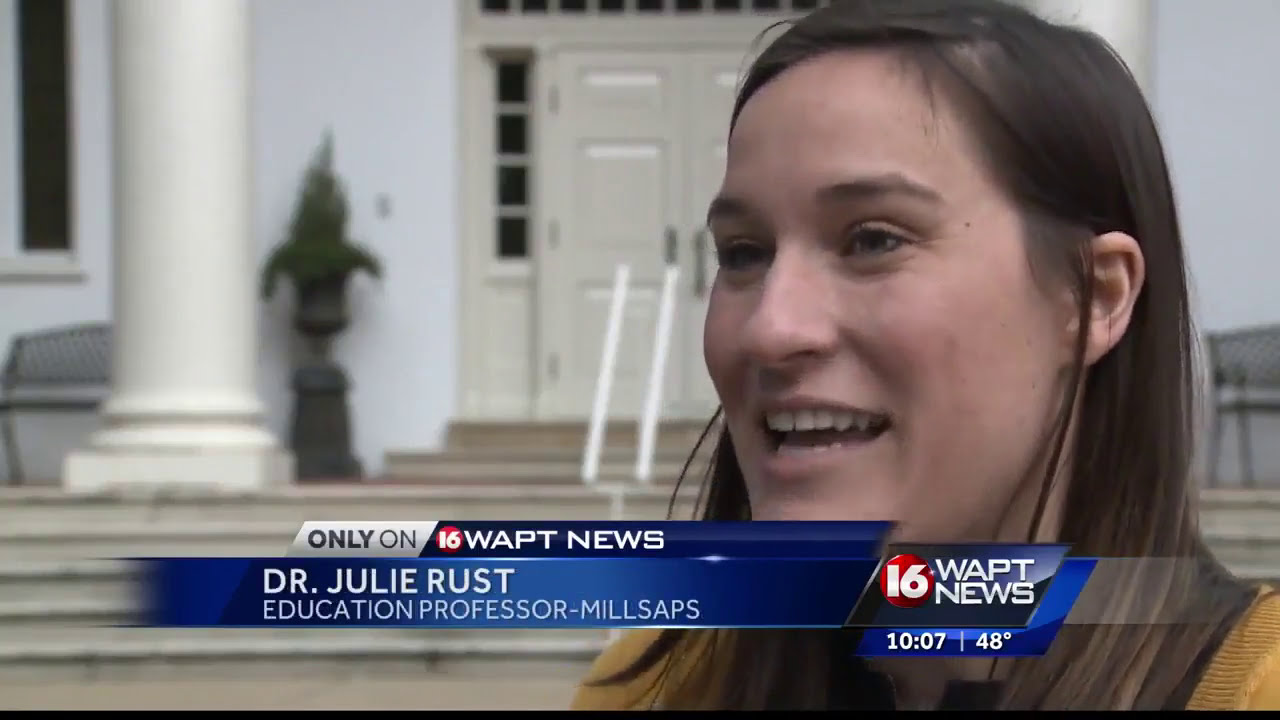The image captures a still from a news broadcast featuring a close-up of a Caucasian woman named Dr. Julie Rust, an Education Professor at Millsaps College. The scene is centered on Dr. Rust, who has shoulder-length, thin brown hair and is wearing a yellow sweater with a possible brown strap over her left shoulder. The background shows a blurred white building with white stairs, columns, and doors, indicating a formal or institutional setting such as a government building or school. A potted plant is also visible near the building's entrance. The news graphic imposed at the bottom of the screen reads, "Only on 16 WAPT News," with her name and title underneath. To the right, the graphic displays the station, "16 WAPT News," the time "10:07," and the temperature, "48 degrees." Dr. Rust is speaking and appears to be engaged in an interview, potentially discussing an educational topic related to her expertise.